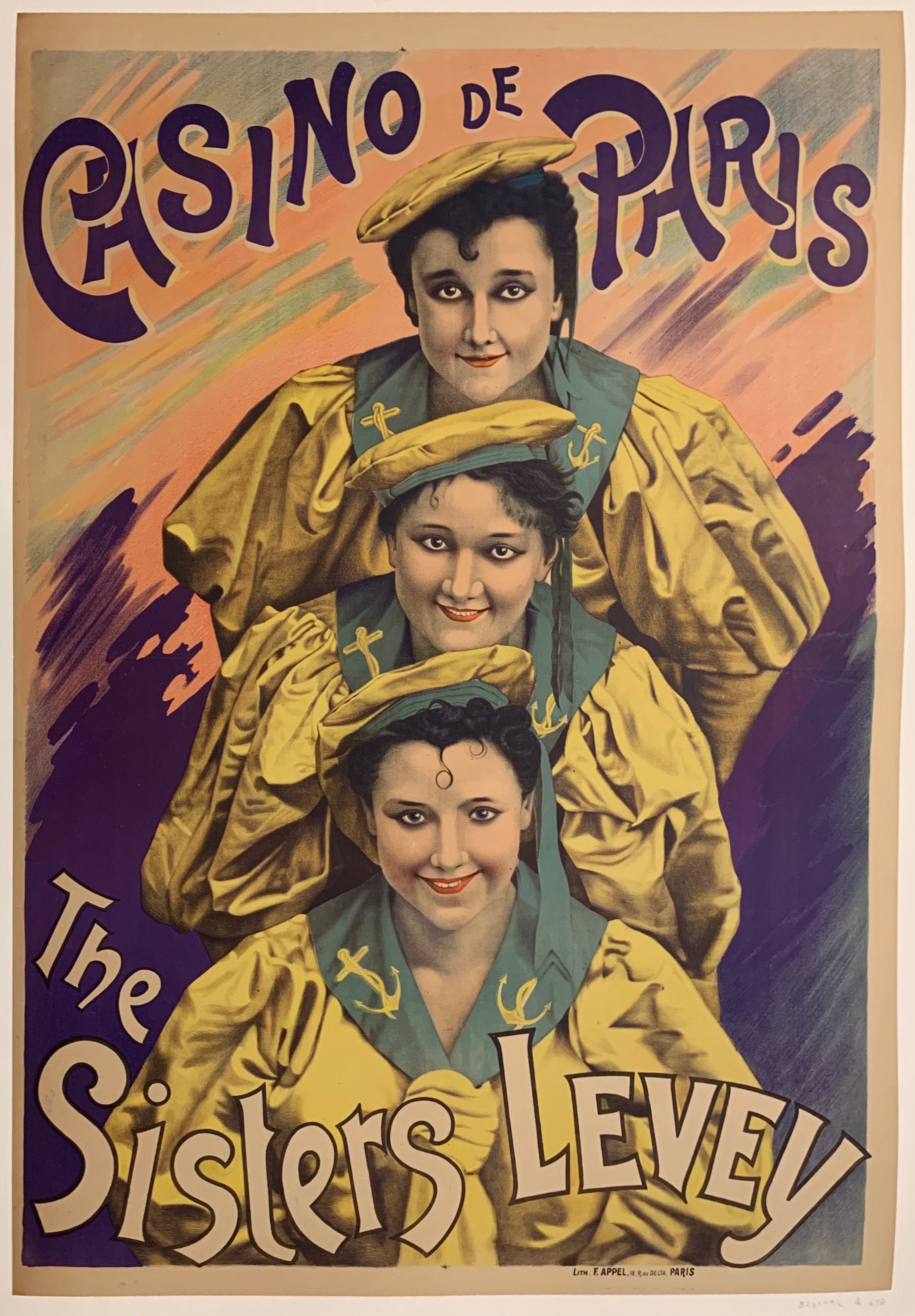The image is a vibrant, colorful poster advertising an event at the Casino de Paris, prominently featuring "The Sisters Levy." Positioned center-frame, the trio of women, apparently sisters, are dressed in striking yellow gowns with teal collars adorned with anchors. They also wear matching yellow and teal beret-like hats, adding to their coordinated ensemble. The women are arranged in a vertical alignment, with one sister at the top, another slightly below her in the middle, and the third sister at the bottom, each head appearing progressively lower. The background features artistic splotches of pink, blue, and purple, with purples becoming more dominant towards the bottom of the image. The poster's backdrop is framed by a light brown border and an additional light gray outer border. The clarity of the image is excellent, revealing every detail in bright, natural lighting. Notably, the words "Casino de Paris" arc gracefully around the top sister's head, with "The Sisters Levy" scripted in blue text at the bottom, highlighting their star billing for this event.